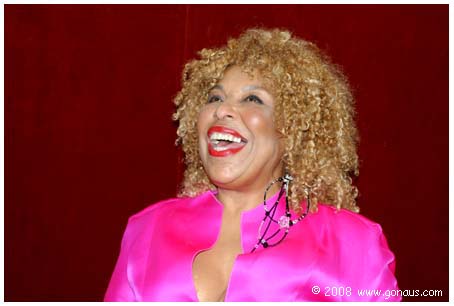A powerful image captures an African-American woman in the throes of an impassioned performance, singing with her mouth wide open and eyes gazing upward toward the ceiling. The focal point is framed from her chest upwards, revealing her attire—a striking, shiny, bright pink top that plunges to reveal her cleavage. Her hair is a cascade of tight, blonde ringlets that frame her face, with a delicate chain cascading from the right side of her hair, flowing down the front of her outfit. Complementing her vibrant outfit, she sports bright pink and red lipstick that emphasize her expressive demeanor. The rich, burgundy red background accentuates the vivid colors of her ensemble. The bottom of the image features the text "2008," though a portion of the website name is illegible.